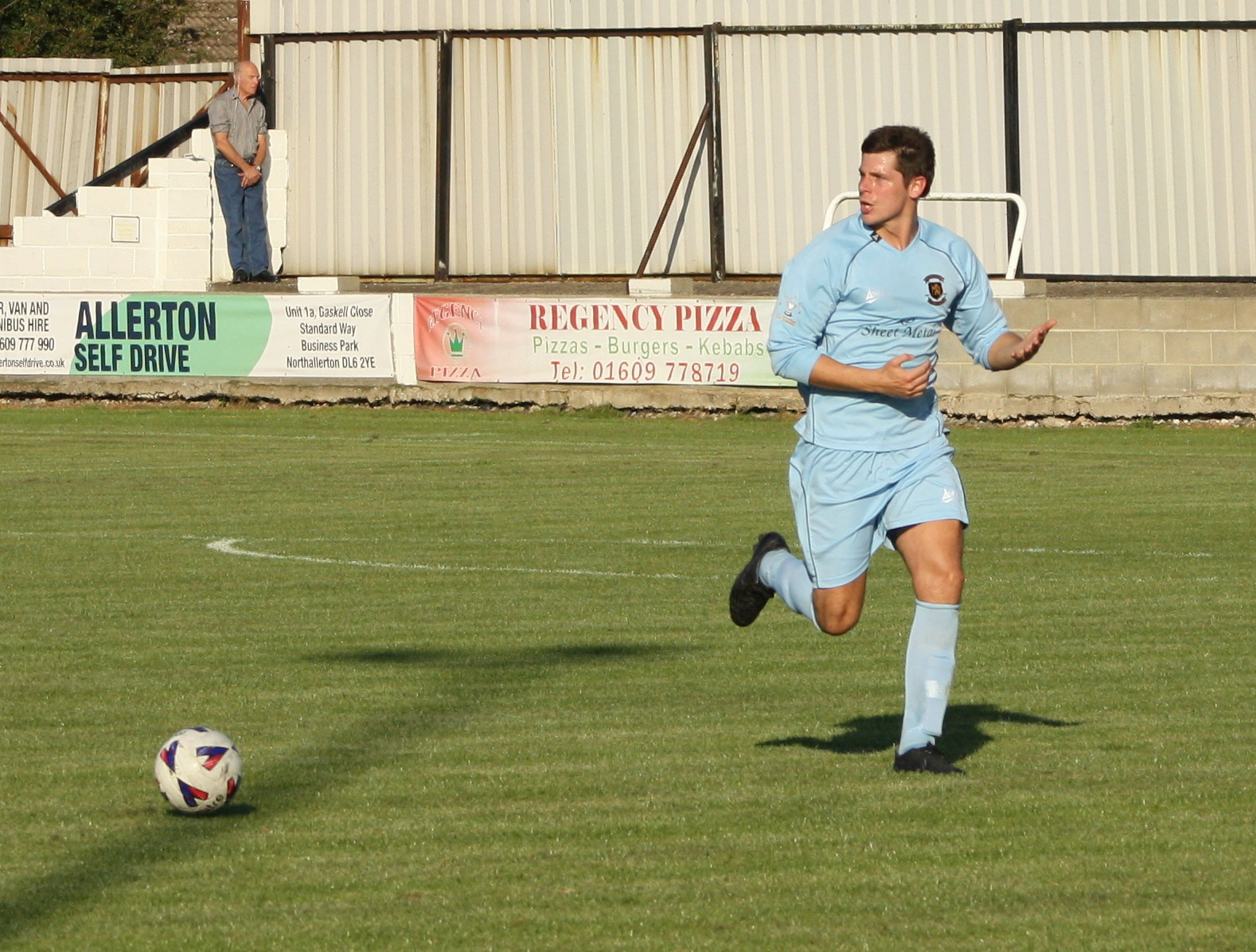In this detailed outdoor daylight photograph, a man with short dark hair and fair skin is captured running on a soccer field. He is wearing a light blue top, light blue shorts, long light blue socks, and black athletic shoes. The player, positioned toward the right side of the image, is in mid-stride, running to the right while his head is turned to the left. His arms are extended forward as if preparing to catch something. About five feet to his left, on the ground, is a soccer ball sporting a white, blue, and red design. 

In the background, an older man, dressed in a gray collared shirt and blue jeans, leans against a concrete wall that lines the edge of the field. Above the concrete wall, there is a taller metal fence supported by a black frame. The wall features various advertisements, including "Regency Pizza" and "Allerton Self Drive, Unit 1A, Gasco Close, Standard Way Business Park, North Allerton DL6 2YE." Further details on the Regency Pizza ad mention "Pizzas, Burgers, Kebabs" along with a contact number, 01609 778719. 

The soccer field is painted with white lines, possibly indicative of the center field circle or goalkeeper zone. To the left of the image, nearer the bottom corner, a shadow cast by a tall pole stretches across the green turf. The setting appears to suggest a practice session rather than a formal game.